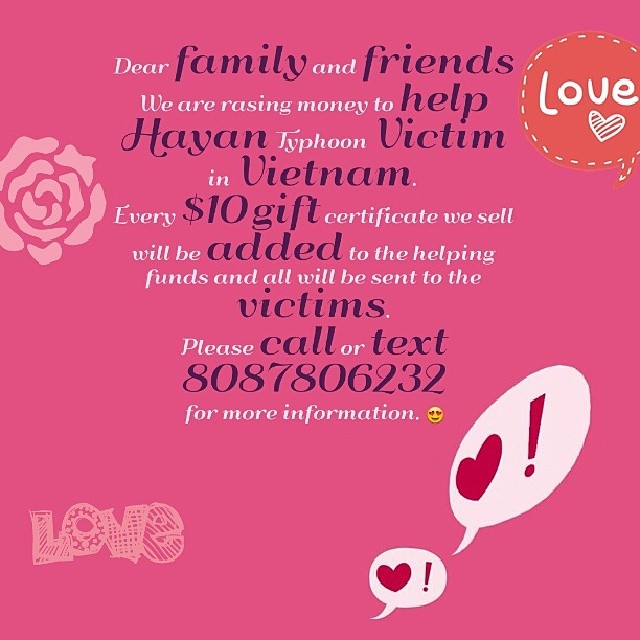This image appears to be an advertisement, possibly seen on social media like Facebook, with the goal of raising money to help Haiyan typhoon victims in Vietnam. The text in the ad alternates between red and dark pink or purple. It reads: "Dear family and friends, we are raising money to help Haiyan typhoon victims in Vietnam. Every $10 gift certificate we sell will be added to the helping funds and all will be sent to the victims. Please call or text 808-780-6232 for more information." 

The background of the ad is completely pink, adorned with various graphics for added visual appeal. In the upper right corner, there is a speech bubble that says "love" with a heart inside it. The upper left corner features a minimalist clip-art outline of a rose. The bottom left corner displays the word "love," written in a sketchy style with unique designs in each letter, such as polka dots in the "O" and stripes in the "E." In the bottom right corner, there are two speech bubbles, one containing a heart and the other an exclamation mark. Additionally, there's an emoji with heart eyes placed next to the contact information for a touch of emotive appeal.